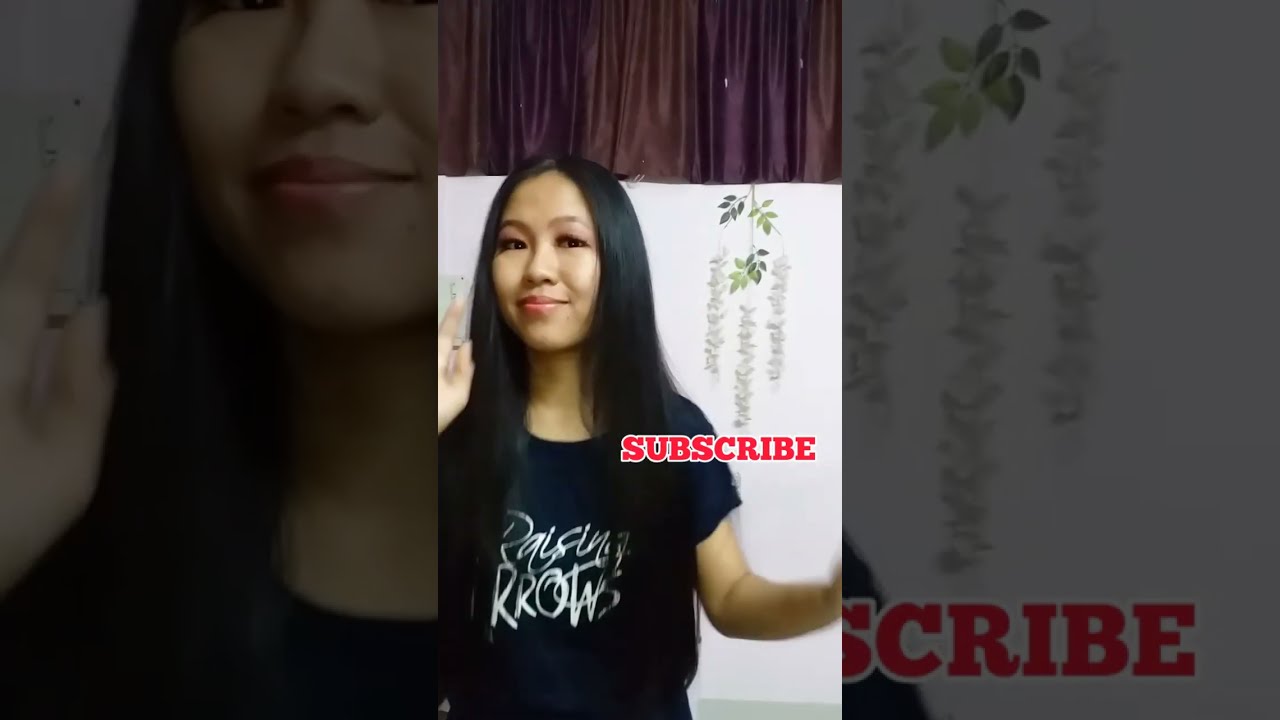In this color photograph taken in portrait mode, a woman with long, straight black hair and prominent cheekbones is depicted smiling softly, her gaze directed slightly to the right. She wears a black t-shirt partially obscured by her hair, but readable white text suggests it might say "Raising" though the exact wording is unclear. Her left arm is slightly raised, contributing to her poised appearance. The background features a white screen adorned with green-leafed tree branches painted to softly descend, accompanied by sporadic white flowers. Above her head, a curtain with alternating brown and purple sections can be seen. Towards her left shoulder, in the image's center, there are bold red letters spelling "subscribe" though it's not perfectly centered. The overall photograph is the central panel of a larger image, flanked on either side by darkened, enlarged portions of the same photograph, creating a framed effect around the central shot.